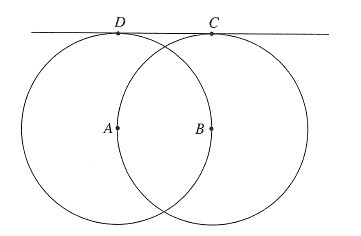The image features a prominent composition consisting of two key elements: a thin horizontal line at the top and two large intersecting circles below it. The circles occupy a significant portion of the image, with their tops just touching the thin line above.

The thin line has two distinctive dots where it meets the tops of the circles. Over the left circle, there's a dot with the letter "D" positioned near it, and over the right circle, there's a dot with the letter "C" below it at the intersection point with the line.

Within the intersecting circles, additional labels are visible. In the left circle, a dot marked with "B" is situated at the middle-right side, which coincides with the center of the right circle. Furthermore, the letter "A" is placed in the middle of the left circle, extending into the left side of the right circle. This detailed labeling and intersection suggest a diagram likely depicting a Venn diagram or a similar conceptual illustration.